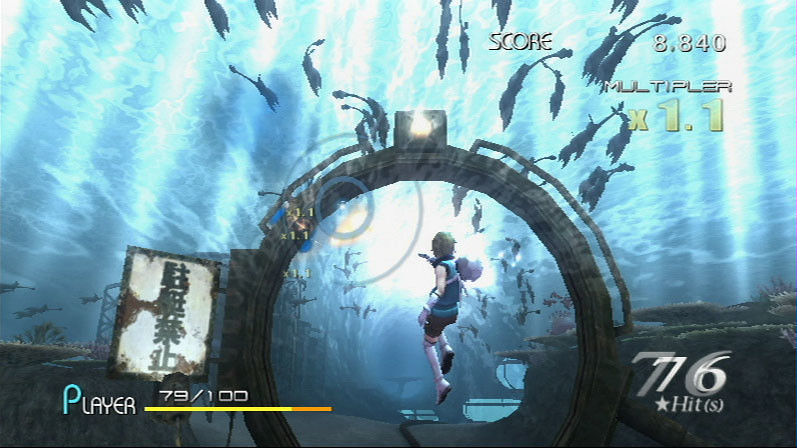Screenshot of an underwater-themed Japanese video game showing a dramatic moment. On the left side of the image, there is Japanese text possibly indicating game instructions or narrative elements. The centerpiece of the scene is a grand gateway, surrounded by a flurry of fish swimming towards it, adding to the immersive underwater atmosphere. On the lower left side of the image, gameplay statistics are visible: "Player: 79/100" indicating the player's current status or level, accompanied by a health bar showing remaining health. In the bottom right corner, "76 Hits" reflects the player's recent performance. The upper right corner displays a score of "8840" and just beneath it, a multiplier of "x1.1". At the heart of the image, the player's character, clad in a detailed scuba outfit, is poised and ready to face underwater challenges. The entire scene is beautifully rendered, capturing the fantastical elements of an underwater adventure.